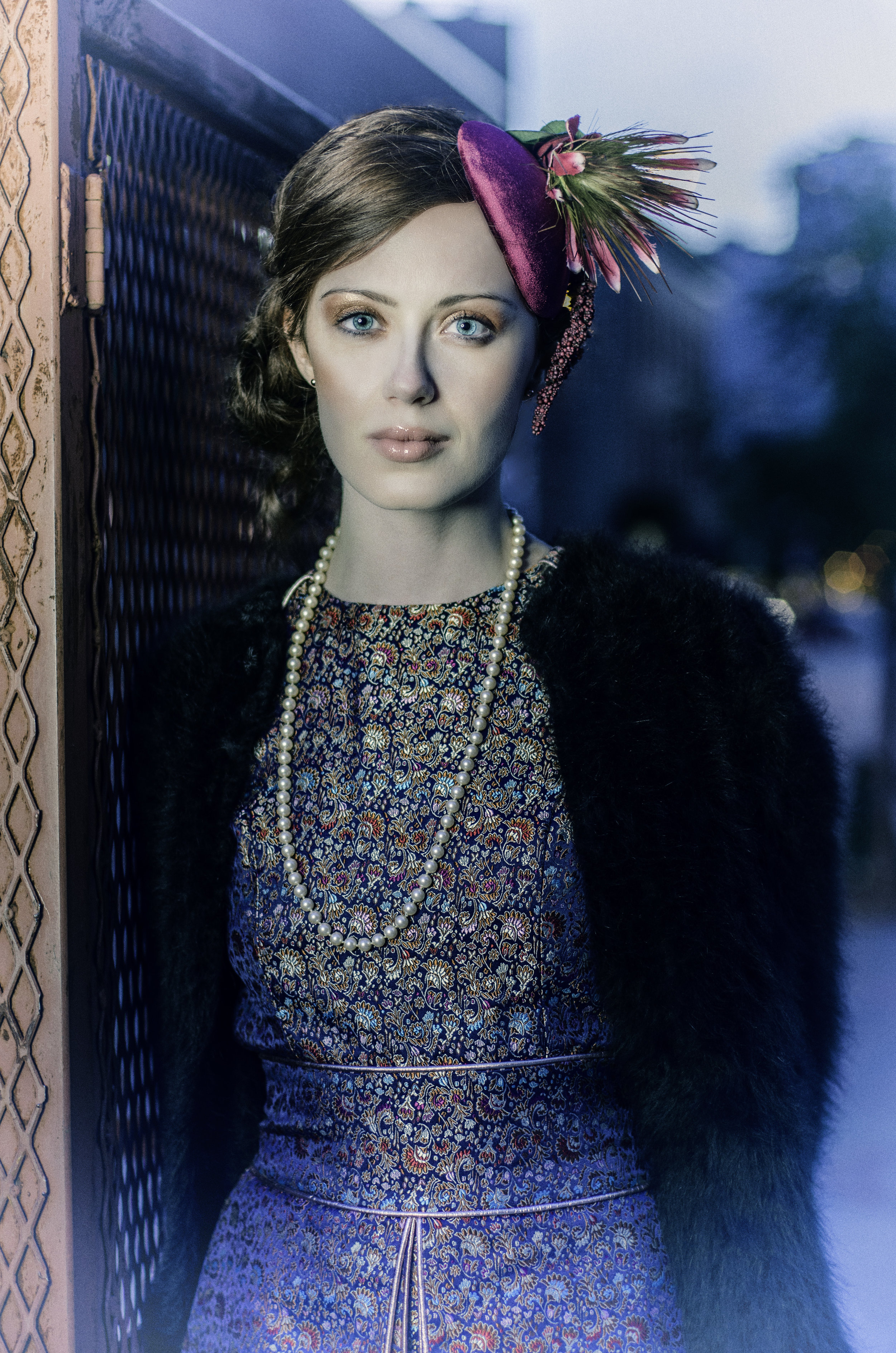This stylized photograph captures a striking portrait of a woman with bright blue eyes, leaning against a metallic gate with a background that is blurred, possibly showing buildings and trees. She has her hair pulled back, adorned with a purple headdress featuring flowers or feathers on the right side. The woman wears a flapper-style outfit reminiscent of the 1930s, including a fur coat over a dark, intricately textured dress with patterns resembling shells or sea creatures in colors like orange, blue, white, and red. She also wears a long pearl necklace. Her complexion is white, and the backdrop, suggestively taken at dusk or dawn, enhances the vintage, stylized aura of the image. The lighting and possible post-processing have given the photo an aged look, reminiscent of a colorized black and white photograph. The scene seems to be a cityscape with blurred light sources, adding to the overall atmospheric and somewhat timeless quality of the image.